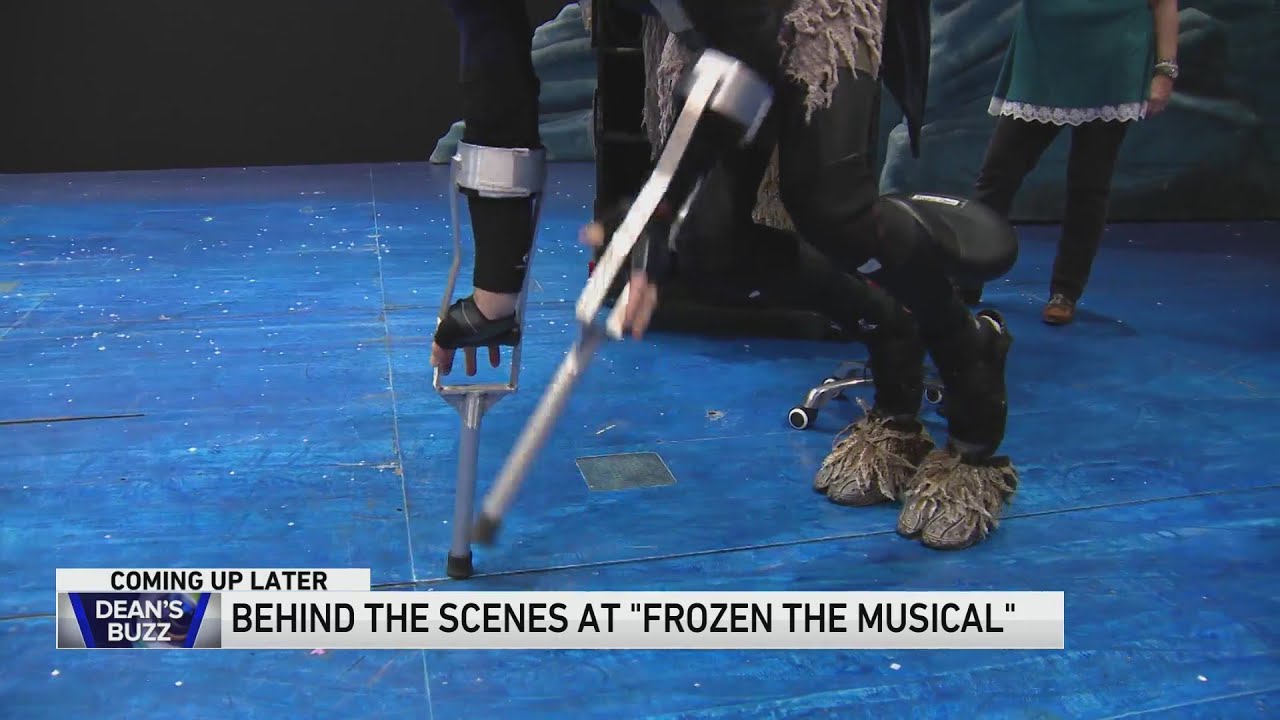This screenshot from a TV or online show, labeled at the bottom with "Dean's Buzz coming up later: Behind the Scenes at Frozen the Musical," features a blue floor that appears somewhat like painted cardboard. Dominating the foreground is a figure dressed in black, seen only from the waist down, walking with crutch-like objects and wearing hoof-type footwear, likely portraying the reindeer character from Frozen. In the background, to the top right, another person is visible, also shown from the waist down, wearing a green dress over pants with lace trim, resembling a townsfolk costume. The scene offers a detailed glimpse behind the scenes of the musical production.